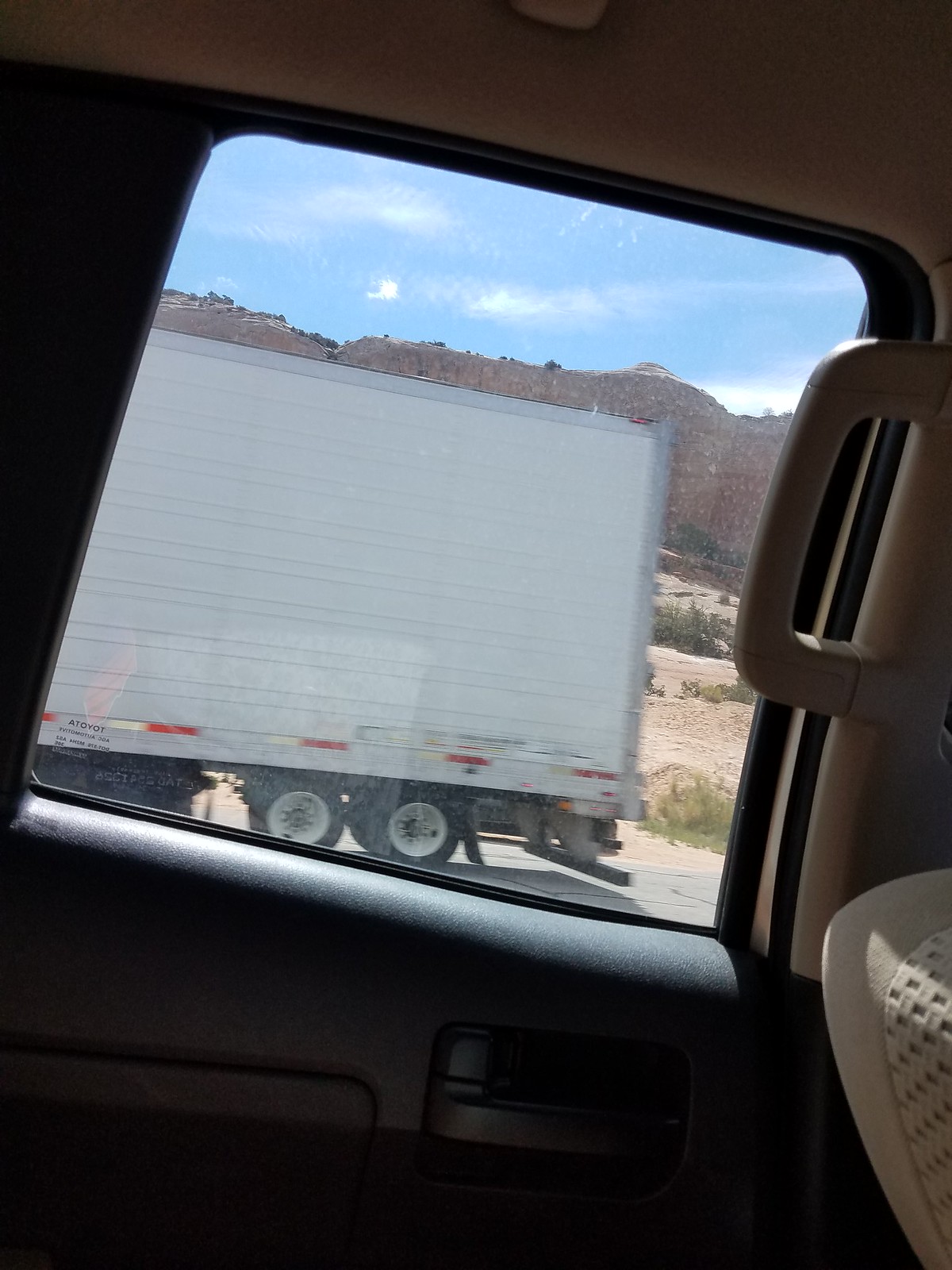This photograph, taken from inside a vehicle with a black and cream interior, captures a desert landscape through the window. The camera perspective, likely from the back seat, reveals the gray, slightly cracked highway alongside a partial view of a semi-truck's white trailer, displaying its rear wheels. The barren surroundings feature expansive stretches of brown dirt and gravel, dotted with small patches of green shrubbery. In the background, distant dark brown hills or small mountains rise against a backdrop of a blue sky adorned with wispy clouds. The scene unfolds at a slight rightward angle, emphasizing the vastness and arid beauty of the desert terrain, possibly located in the western part of the country.